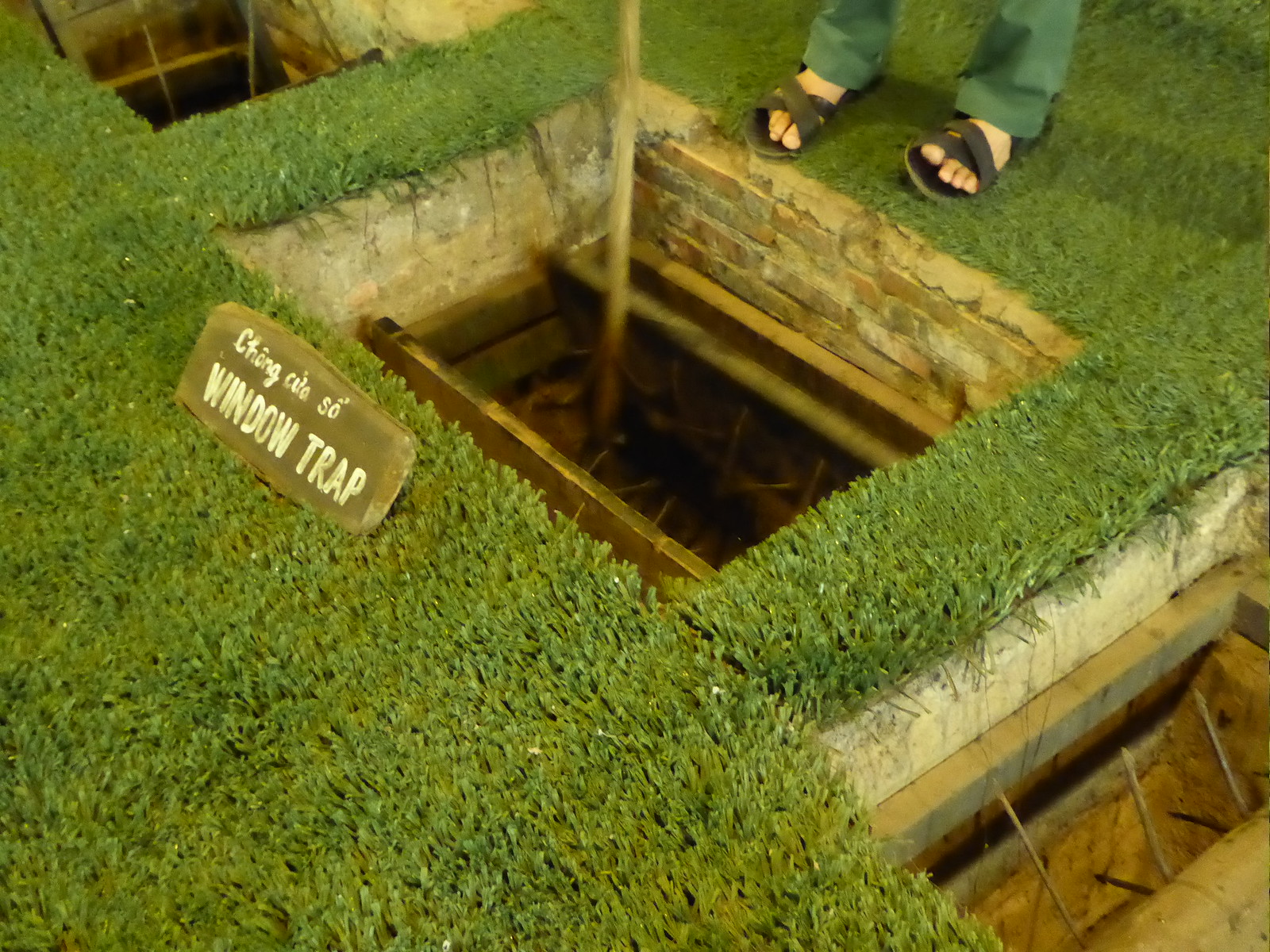This detailed photograph depicts a man standing on artificial green turf, partially over a square hole in the ground labeled as a "window trap." His attire features dark green pants and brown sandals, revealing only his legs up to mid-calf. The focal point of the image is the trap door in the center, bordered by bricks and artificial grass. Within the trap, there is a metal pipe or stick being manipulated by the man. There are two other similar traps positioned diagonally—one in the bottom right and one in the top left of the frame—each with wooden rods and spikes, suggesting they can rotate. A sign near the top left trap reads "Chong CSO" and "Window Trap" in English. Additional elements include fake grass, bricks forming part of the background, and signage that might relate to historical or educational exhibits. The vivid colors ranging from the green turf, brown and gray brick, to the peach hue of the man's visible skin, contribute to the image's overall detail. The setup appears to resemble a museum exhibit focused on showcasing historical or war-related traps.